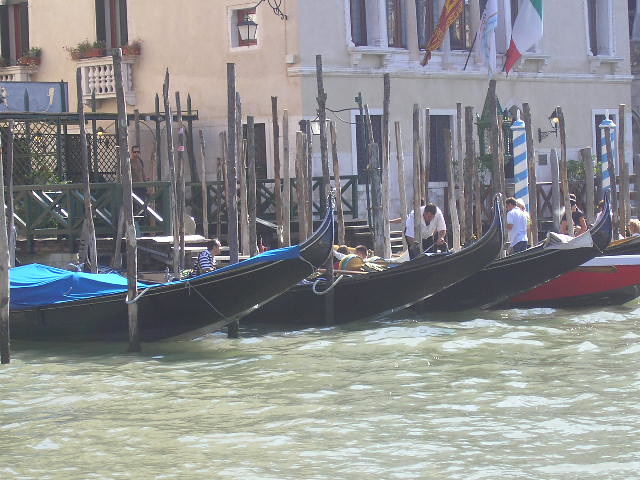This image depicts a bustling dock in Venice, Italy, characterized by its signature narrow canals and murky green waters. On the waterway, four traditional Venetian boats, likely gondolas given their black exteriors and uniquely pointed, upturned bows, are securely tied to tall, brown wooden posts, ensuring they remain stationary. Each boat gleams with distinct details; one is partially covered with a blue tarp, while another contains a variety of brown wooden items or decorations. 

The dock itself appears rudimentary, with its simple construction complementing the scene's historical ambiance. Surrounding the boats, several people can be observed, suggesting activity and preparation. Notably, a gentleman in a blue and white striped shirt sits calmly in one boat, while another man, in a white t-shirt, bends over to secure a rope, accompanied by two unseen individuals. Further along, a red, black, and white boat hosts a man standing with his back to the camera, donned also in a white t-shirt.

In the background, the scene is framed by elegant Venetian architecture—a large tan stone building adorned with intricately designed awnings and windows, punctuated by light blue and white striped posts and an Italian flag fluttering nearby. The overall composition captures the quintessential charm and activity of a Venetian canal dock.